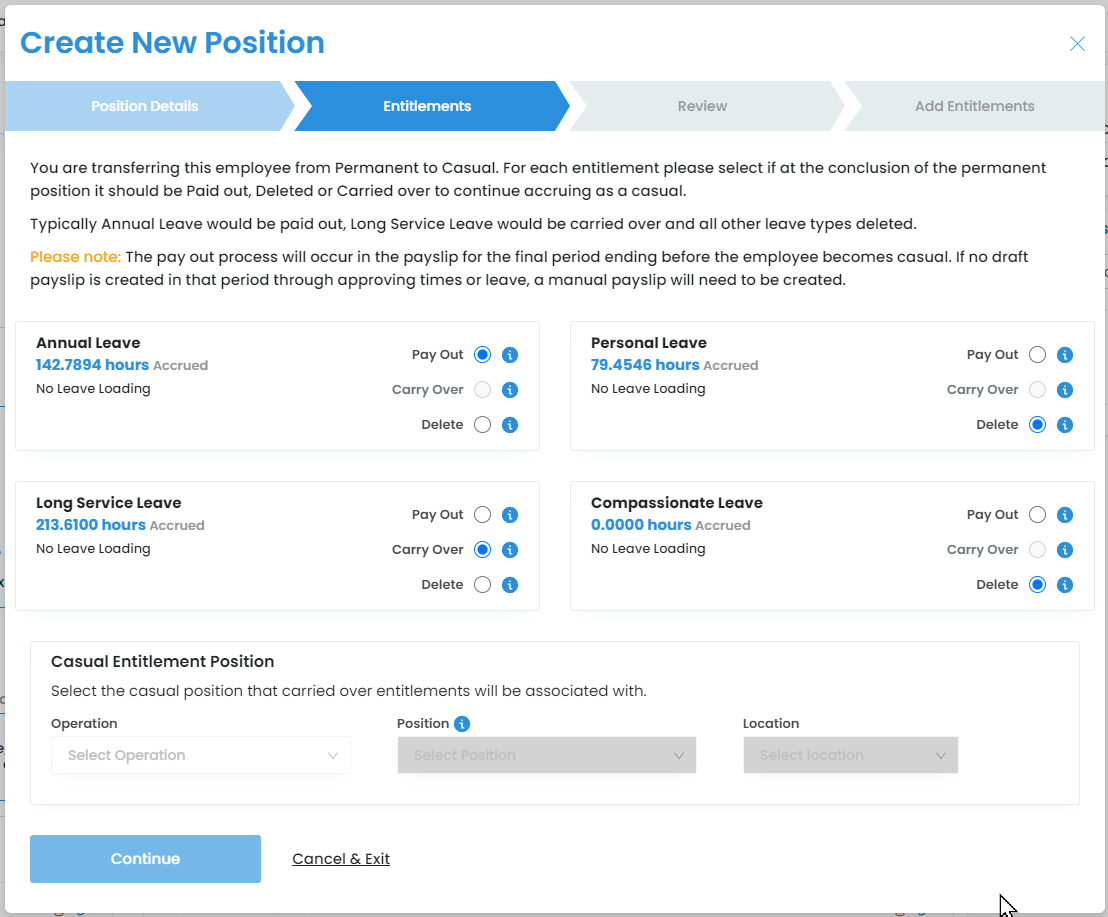The screenshot depicts a digital interface in the middle of a multi-step workflow titled "Create New Position," highlighted in blue at the upper left-hand corner. The workflow is divided into four sequential sections: Position Details, Entitlements, Review, and Add Entitlements. The first section, Position Details, is marked as completed, while the second section, Entitlements, is currently active, highlighted in dark blue. The remaining sections, Review and Add Entitlements, are grayed out, indicating they have yet to be addressed.

Directly beneath the workflow indicator, there is a block of text in black font consisting of three paragraphs, detailing the process of transferring an employee from a permanent to a casual position. 

The main part of the interface is organized into four sections. On the lower left, the "Annual Leave" section shows accrued leave time of 142.7894 hours with no leave loading, accompanied by three radio button options: Payout, Carryover, and Delete, with Payout currently selected. Below it, the "Long Service Leave" section presents the same radio button choices, with Carryover selected.

On the right-hand side, two additional sections follow a similar format. The "Personal Leave" section has the Delete option selected, as does the "Compassionate Leave" section below it.

At the bottom of the interface, there is a section titled "Casual Entitlement Position," which is currently grayed out, signifying that it is not yet actionable. Below this section, there are two navigational options: a button to continue with the workflow and a link to cancel and exit the process.